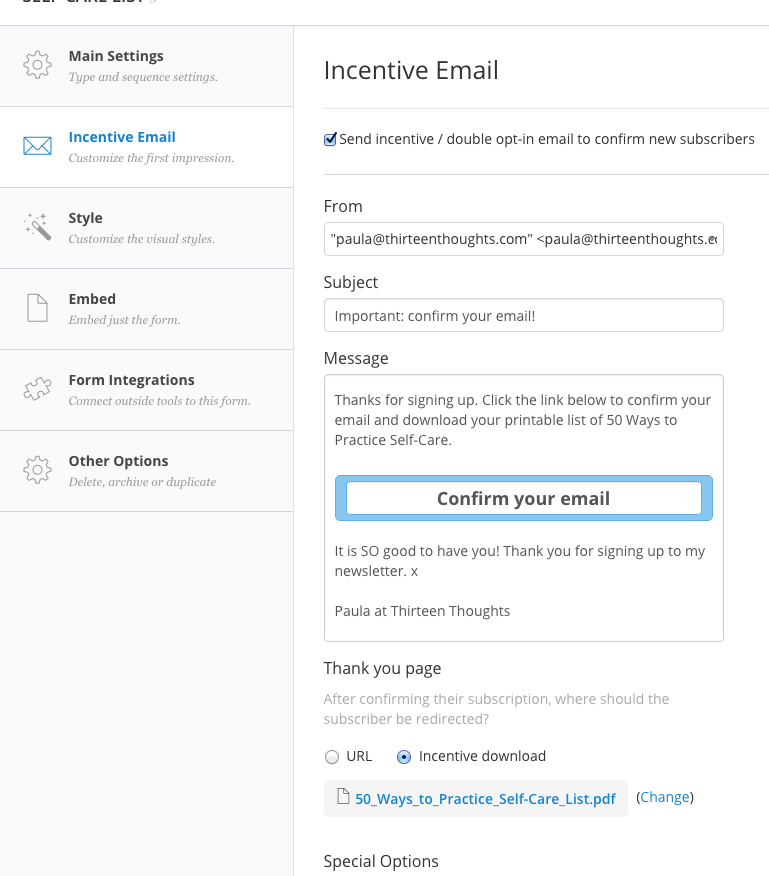This detailed caption describes an online email settings page consisting of two vertically oriented columns. 

On the left, occupying about 35-40% of the image width, is a segmented panel with a light gray background. The panel, bordered only at the top and right, is divided into six fields. The top field, marked "Main Settings" in bold, includes smaller italicized text reading "Type and sequence settings" alongside a gear icon. The second field, highlighted in white with blue text, is labeled "Incentive Email" and subtitled "Customize the first impression" with an envelope icon. The remaining four fields revert to the original gray background and are labeled "Style," "Embed," "Form Integrations," and "Other Options," each accompanied by a relevant icon (a magic wand, a folded paper, a puzzle piece, and another gear).

On the right, the column, constituting about 55-60% of the image width, features a white background. The heading "Incentive Email" is displayed in the upper left. Below, the first section includes a checkbox labeled "Send incentive/double opt-in email to confirm new subscribers," bordered above and below by thin lines. The following fields provide spaces for "From" (pre-filled with "paula@13thoughts.com" in quotation marks and triangular brackets), "Subject" (filled with "Important: Confirm your email!"), and "Message." The "Message" field is almost square, with a bold "Confirm your email" call-to-action button in the middle, outlined in light blue. Below, the "Thank You Page" section contains only the header and two lines of text, followed by two radio buttons labeled "URL" (unchecked) and "Incentive Download" (checked).